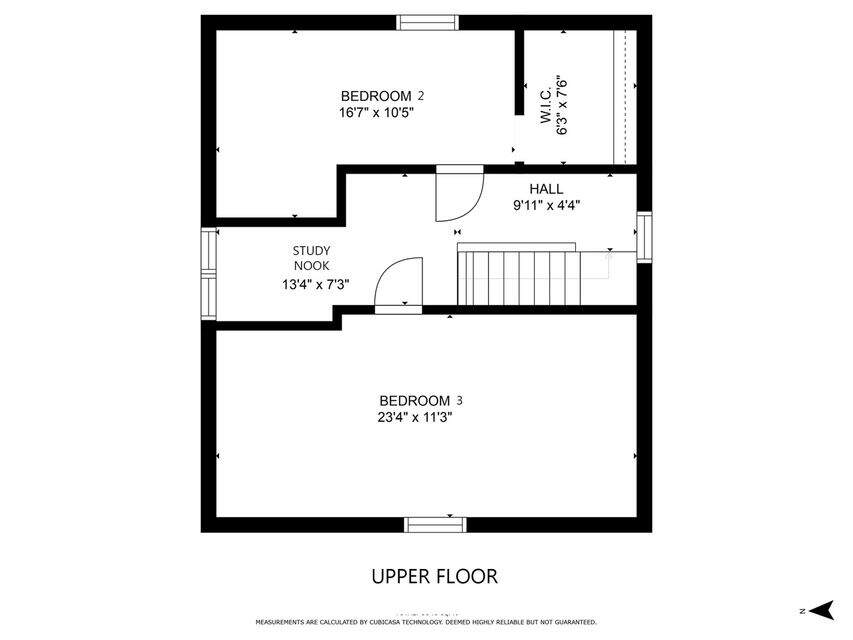This architectural graphic illustrates the floor plan for an upper floor, specifically detailing Bedroom 2 and ancillary spaces. Bedroom 2 measures 16 feet 7 inches by 10 feet 5 inches and features an attached walk-in closet sized at 6 feet 3 inches by 7 feet 6 inches. This room is accessible via a door and includes a window. Upon ascending from the central staircase, a hallway provides ingress to both Bedroom 2 and Bedroom 3. The third bedroom is notably larger, spanning 23 feet 4 inches by 11 feet 3 inches, with one window but lacking any closets. Adjacent to the staircase is a designated study nook that measures 13 feet 4 inches by 7 feet 3 inches and is illuminated by several windows. A footnote at the bottom mentions that the requirements are calculated using CUBJ CASA technology, which is regarded as highly reliable but not guaranteed. The lower right corner of the graphic features a north arrow, indicating that north is oriented to the left.